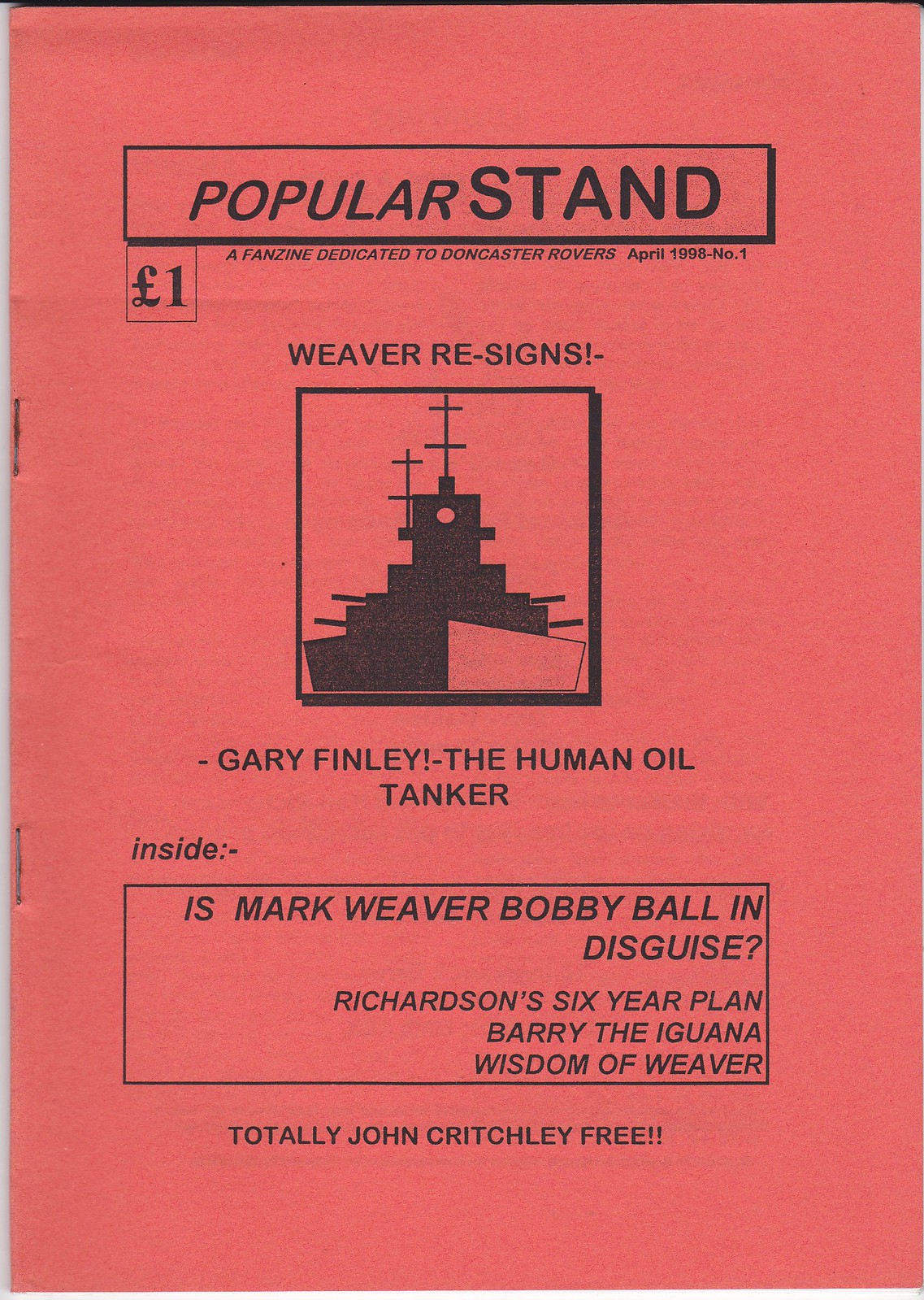The image features the cover of a rust-colored brochure, resembling construction paper, with black print. The header reads "Popular Stand" within a rectangular black border, indicating it's a fanzine dedicated to Doncaster Rovers from April 1998, issue number one, priced at one pound. Below the header, there's a bold announcement, "Weaver Re-signs," accompanied by a central square illustration that appears to be a crude drawing of an oil tanker or battleship. Directly beneath the illustration is the caption, "Gary Finley, the human oil tanker." Additional details listed on the cover include intriguing teasers such as "Inside: Mark Weaver, Bobby Ball in disguise, Richardson's six-year plan, Barry the Iguana, Wisdom of Weaver." At the bottom of the cover, the text asserts "Totally John Critchley Free." The brochure is fastened with two staples, suggesting a modest number of pages.